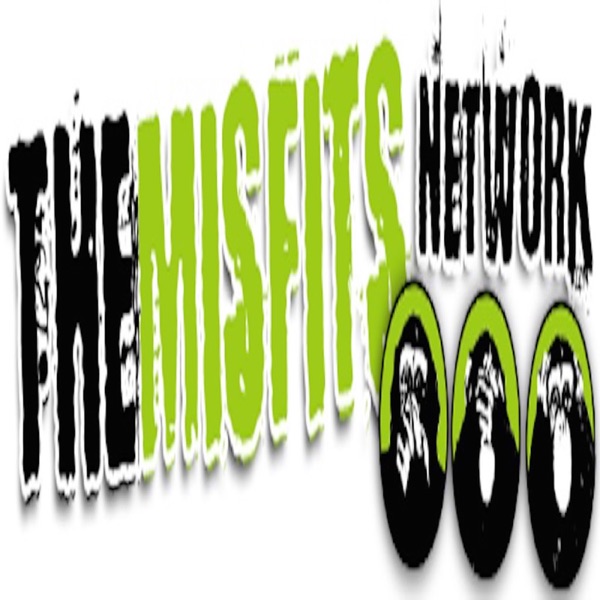The image features a distorted and stylized logo set against a white background, reading "The Misfits Network." The text "THE" is in all caps and black, stretched out and prominently displayed. "MISFITS" is rendered in lime green, all capitalized, with a font reminiscent of the punk band from the 80s and 90s, evoking a distressed, horror-like aesthetic. "NETWORK," also in all caps but smaller and in black font, is positioned to the right. Below the text are three oval images featuring black and white monkeys on a green background, each in a different pose symbolizing the "See No Evil, Hear No Evil, Speak No Evil" motif: one monkey covering its eyes, another covering its ears, and the third covering its mouth.